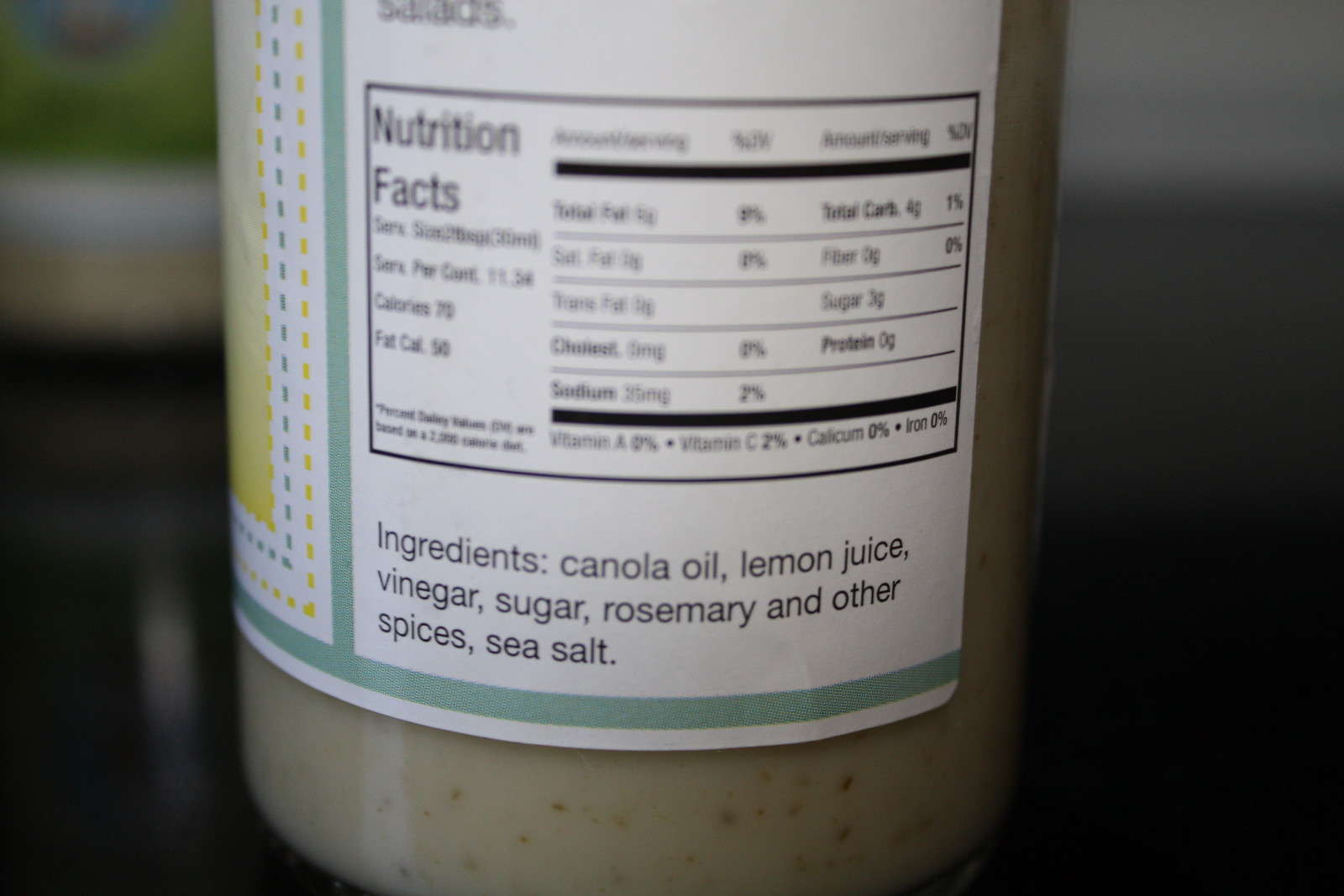The image features a glass jar of food product, likely a type of sauce, that is white or off-white with brown speckles. The jar is positioned on a glossy black surface that reflects some light. In the blurred background, there is an indistinct tan and green object located in the back left corner. The focus of the image is on the jar's white label, which has an aquamarine border accented with yellow and aquamarine designs. The label details the ingredients, listing canola oil, lemon juice, vinegar, sugar, rosemary, other spices, and sea salt. Additionally, the label provides nutritional information, including a serving size of two tablespoons, containing 70 calories, with 50 of those calories coming from fat, although the rest of the nutritional details are too blurry to discern.